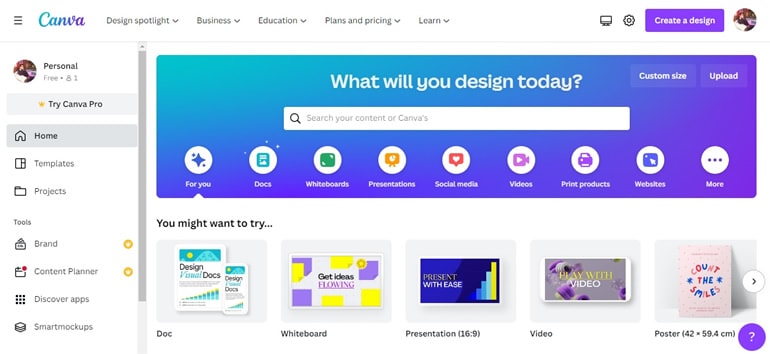The image depicts a Canva web page showcasing its interface. On the left-hand side, a vertical navigation menu lists various options, starting with a profile picture indicating a free account status subscribed under "Personal." The free account is emphasized with a gray rectangle featuring a gold star and the text "Try Canva Pro" prominently displayed in black.

The menu includes:
1. **Home**: Highlighted with a dark gray background and bold black text.
2. **Templates**: Represented by a web page icon divided into sections.
3. **Projects**: Shown by a folder icon.
4. **Tools**: A new section containing various icons, including a thought bubble for "Brand," an orange circle representing "Brand," and additional tools like "Content Planner," "Discover Apps," and "Smartphone Mockups".

On the main canvas, a central text in bold white reads, "What will you design today?" accompanied by a magnifying glass icon in a search bar that prompts users with "Search your content on Canva Canvas."

At the top center of the page, there's a horizontal menu with buttons for "Design spotlight," "Business," "Education," "Plans and Pricing," and "Learn," each followed by a black drop-down arrow. On the far right, there are additional icons:
1. **Device Toggle**: Indicates switching between mobile and desktop view.
2. **Settings**: Represented by a gear icon.
3. **Create a Design**: A rectangular button with a purple background and pink text.

The web page also features various content categories depicted by square icons, each with specific imagery and color:
1. **For You**: A blue icon featuring three diamonds.
2. **Docs**: A teal document icon.
3. **Whiteboards**: A green icon with writing lines.
4. **Presentations**: An orange TV-like icon.
5. **Social Media**: A red square with a white heart.
6. **Videos**: A purple video camera icon.
7. **Print Projects**: A purple printer icon.
8. **Websites**: A blue icon with an arrow and dot.

At the bottom, additional sections like Docs, Whiteboards, Presentations, Videos, and Posters are indicated with corresponding pictographic representations.

The overall organization and color scheme enhance user navigation, making it intuitive and visually engaging.